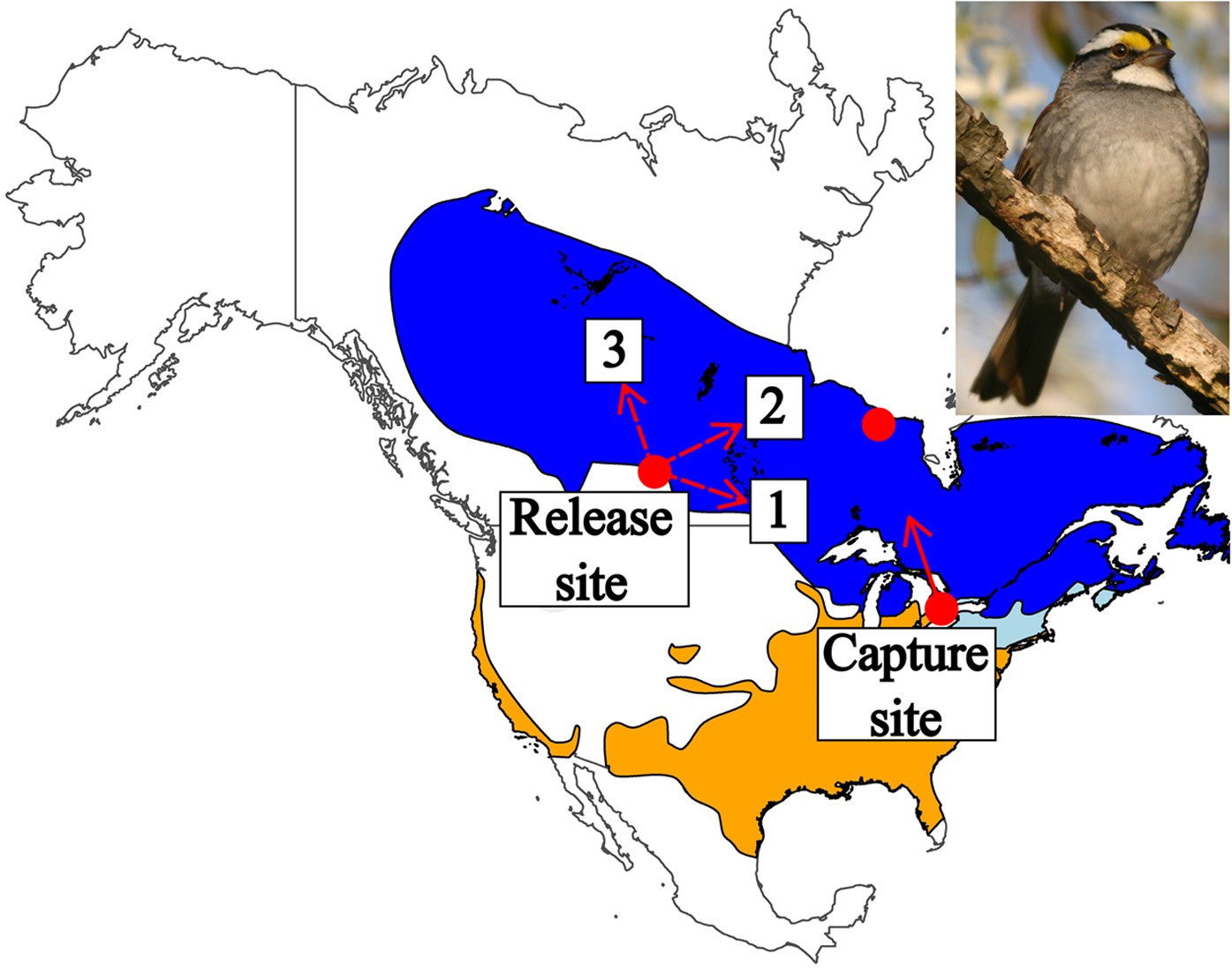This image features a detailed map highlighting the United States, Canada, and Mexico. The map displays various shaded regions: the majority of Canada and some parts of the northeastern United States are covered in a swooping blue area, while orange highlights portions of the East Coast, California, Texas, and New Mexico in the United States. Near the center of Canada, three sites are marked with red arrows pointing to numbers 1, 2, and 3 inside a white square, annotated as "Release Site." Additionally, a "Capture Site" marked with red is located towards the bottom right of Canada. 

In the top right-hand corner of the image, there's an illustration of a bird perched on a branch. The bird has a gray body with distinctive black-and-white stripes across its head, white under the neck, yellow above the eyes, and black and yellow tail feathers. Behind the bird, flowers and leaves are faintly visible, adding a natural background element to the image. This image appears to depict the capture and release points for the bird in question, with the three release sites positioned primarily in the middle regions of Canada.